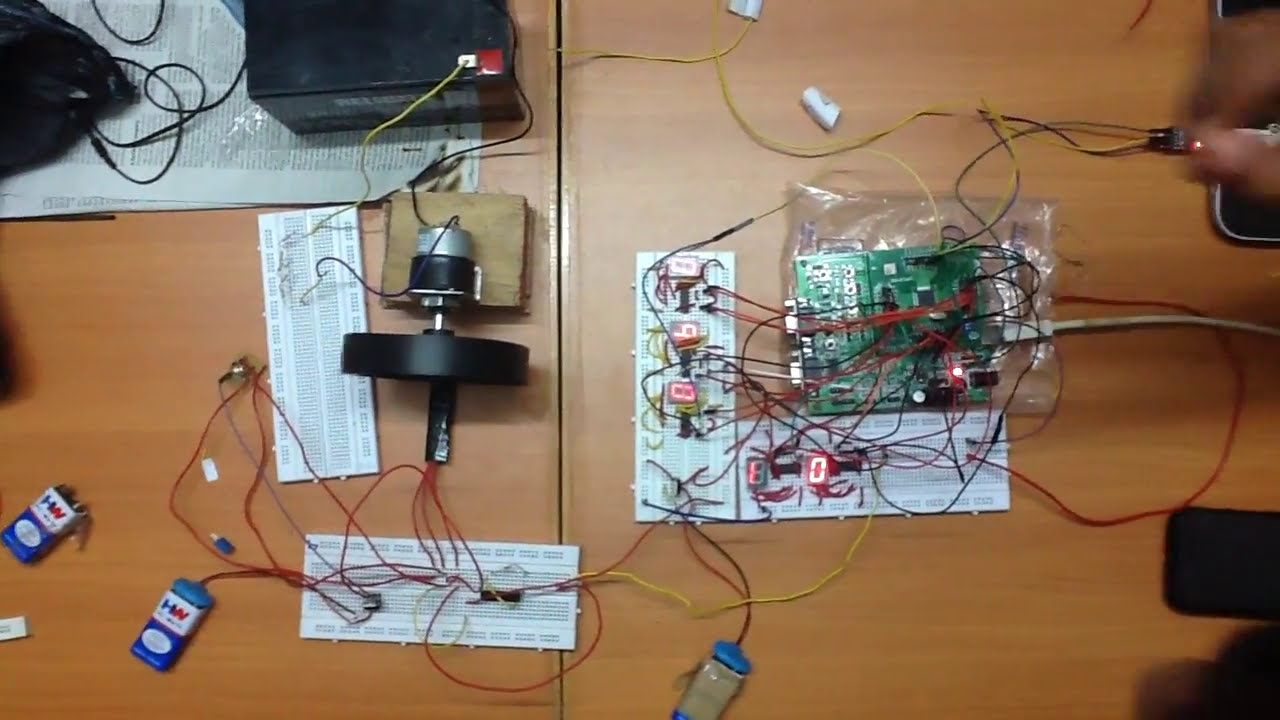An overhead view of a cluttered table reveals a scene of intense electronic repair and assembly, reminiscent of a tech workshop. The table is strewn with numerous black and red cords, white breadboards, and a variety of batteries, some connected and others loose. Centered on the wooden desk area, which resembles a school or office setting, are pieces of disassembled electronic devices, possibly including an alarm clock or a unit with a VCR-like appearance. A green circuit board with a glowing red light, numerous LEDs showing numbers like 09810, and a motor or black wheel connected to a smaller cylinder are evident. To the right, two fingers hold a cord beside a cell phone, a plastic bag filled with new connectors, and a screwdriver indicating ongoing repair or assembly work. Instructions or newspapers are partially buried under the tangle of wires, hinting at a meticulous but chaotic technical endeavor.